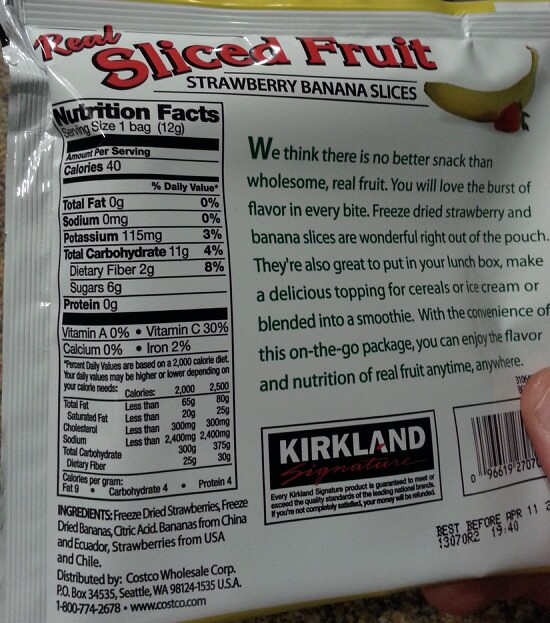In the image, there's a package of fruit slices prominently displayed, showcasing its back side. In the lower right-hand corner, a thumb and part of a finger are visible, holding the bag. The bag features red and black text that reads "Real Sliced Fruit" and "Strawberry Banana Slices." The package also displays the nutrition facts and a descriptive blurb in green lettering. 

The blurb states: "We think there is no better snack than wholesome real fruit. You will love the burst of flavor in every bite. Freeze-dried strawberry and banana slices are wonderful right out of the pouch. They're also great in your lunchbox, make a delicious topping for cereals or ice cream, or blend them into a smoothie. With the convenience of Omnico packaging, you can enjoy the flavor and nutrition of real fruit anytime, anywhere."

The product is labeled as "Kirkland Signature." The nutrition facts detailed in black lettering reveal: one serving size is a 12-gram bag, which contains 40 calories, 0 grams of fat, 0 grams of sodium, 150 milligrams of potassium (3% DV), 11 grams of carbohydrates (4% DV), 2 grams of dietary fiber (8% DV), 6 grams of sugar, 0 grams of protein, and provides 30% of the daily value for Vitamin C and 2% for iron. It mentions no vitamin A or calcium. Additionally, it provides calorie content per gram: 9 for fat, 4 for carbohydrate, and 4 for protein.

Ingredients listed are freeze-dried strawberries and bananas, with citric acid. The sources of the fruit are noted as bananas from China and Ecuador, and strawberries from the USA and Chile. The product is distributed by Costco Wholesale Corporation, based in Seattle, Washington. They provide a contact number, 1-800-774-2678, and a web address, www.costco.com, all printed in black text.